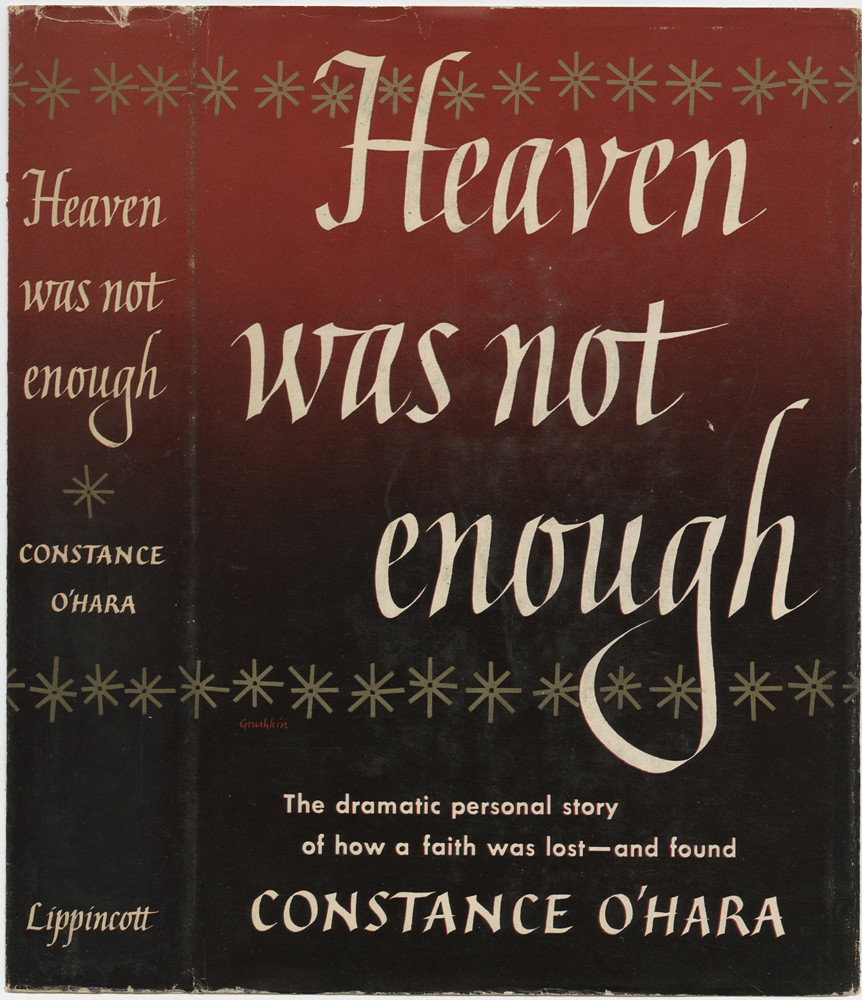The image depicts a slightly weathered book cover showing both the front and the spine of the book, titled "Heaven Was Not Enough" by Constance O'Hara. The cover background features a gradient, transitioning from a vibrant red at the top to a deep black at the bottom. Adorning this gradient background is a line of white drawings near the top and bottom edges, resembling snowflakes or starbursts. The title "Heaven Was Not Enough" is prominently displayed in elegant white script on the front cover, accompanied by the subtitle, "The dramatic personal story of how a faith was lost and found." The spine of the book also bears the title and the author's name, along with the publisher's name, Lippincott.